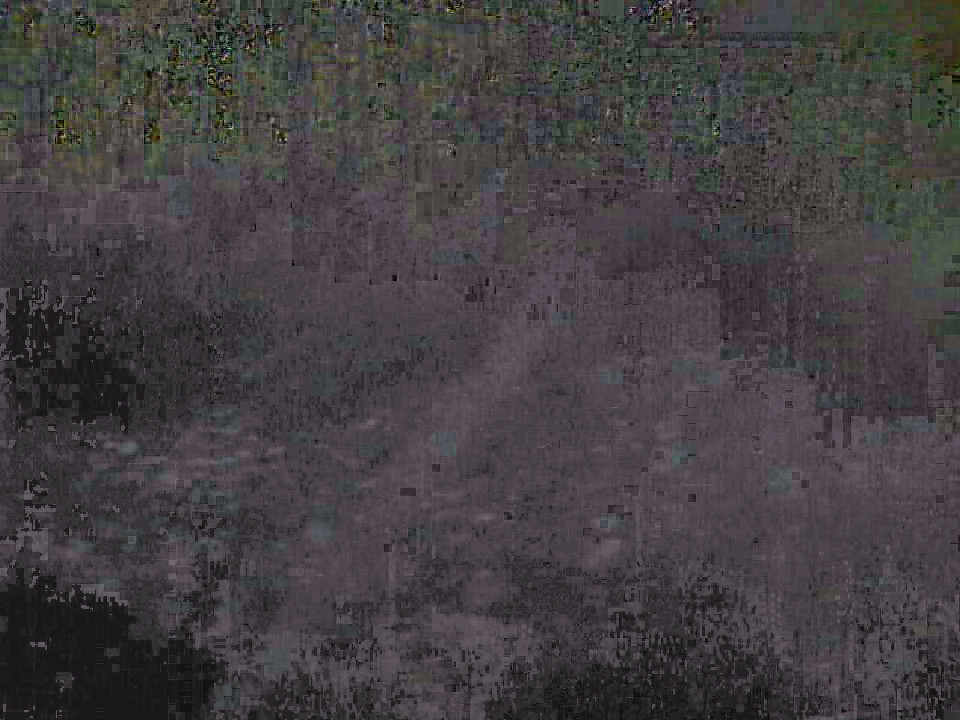The image is heavily pixelated, causing a significant blur that merges the colors together. In the upper section, various shades of green dominate, ranging from a vibrant, bold green to a deeper, darker green, all forming a pattern of small, pixelated squares. The middle portion shifts to hues of purple, with a mix of light purple and numerous dark purple circular shapes scattered throughout. The left-center area features a black background interspersed with green and purple pixelated squares. Finally, the lower left corner is predominantly black, punctuated by more purple pixelated boxes. Overall, the image presents a mosaic of indistinct shapes and blended colors due to the pixelation.